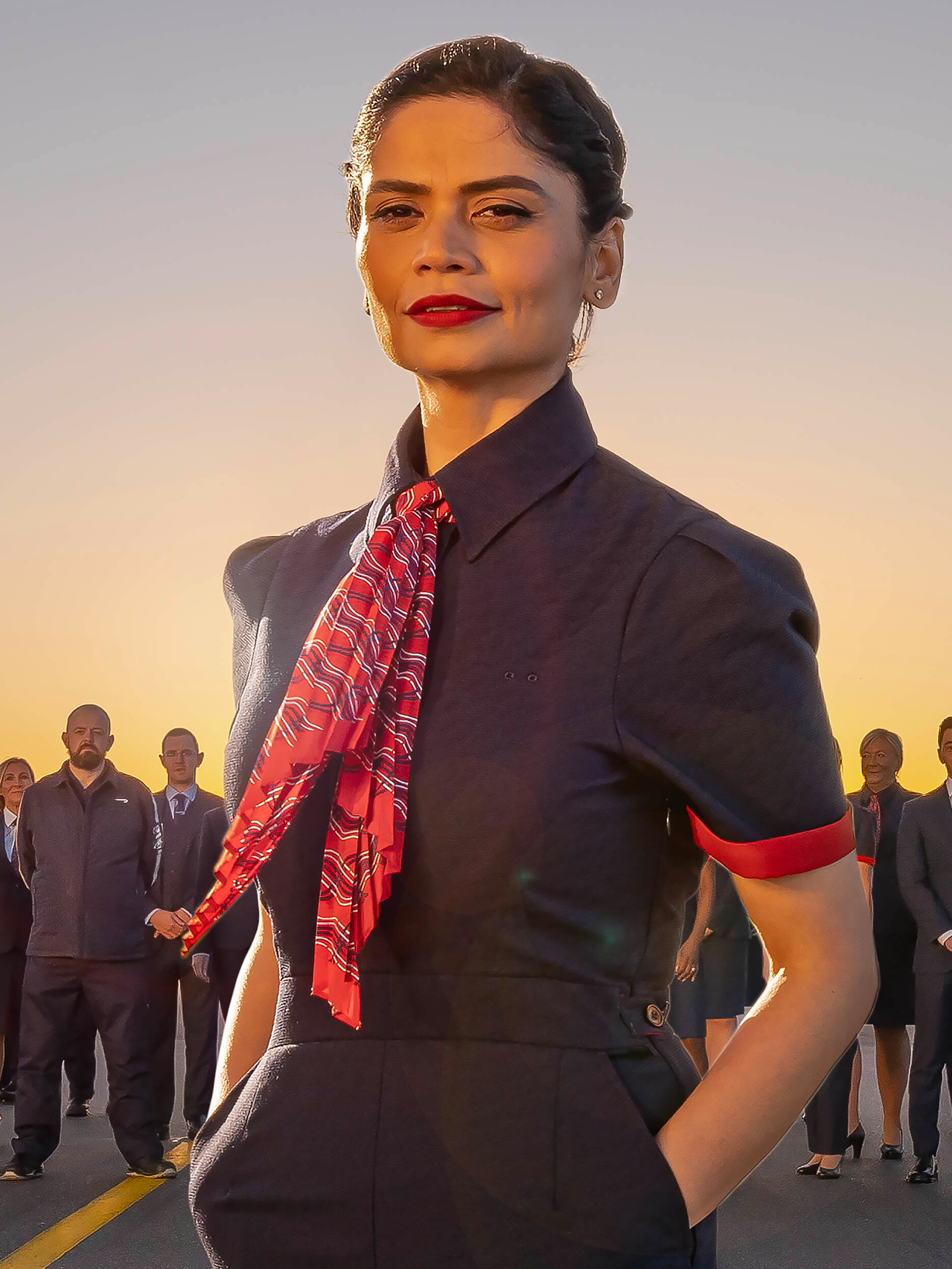The full-color photograph, taken outdoors during daytime, captures an elegantly staged scene intended for artistic and promotional purposes. The backdrop features a clear sky transitioning into an orangish-yellow tint, suggesting the photo was taken around sunrise or sunset. The setting is an asphalt roadway with a distinct yellow line running through it.

The main focus is a young, dark-haired woman centrally positioned in the frame. She is wearing a professional dark blue uniform, likely a flight attendant's outfit, complemented by a red, white, and blue striped kerchief that adds a splash of color around her neck. Her short-sleeved shirt is accentuated with red trim at the sleeve edges, a button on the side, and she pairs it with black pants. She stands confidently with her hands in her pockets, gazing directly at the camera with a slight squint, her hair tied back, and red lipstick highlighting her features.

The background reveals several individuals, all appearing stationary with their hands variously clasped or at their sides. These individuals are dressed in a mix of formal attire including suits, business suits, and coveralls. The scene is set on what appears to be a road or parking lot, evidenced by the flat, gray surface and the yellow dividing line. The sky above them transitions from a light blue to a vibrant orange and pink, adding a dramatic and serene atmosphere to the image.